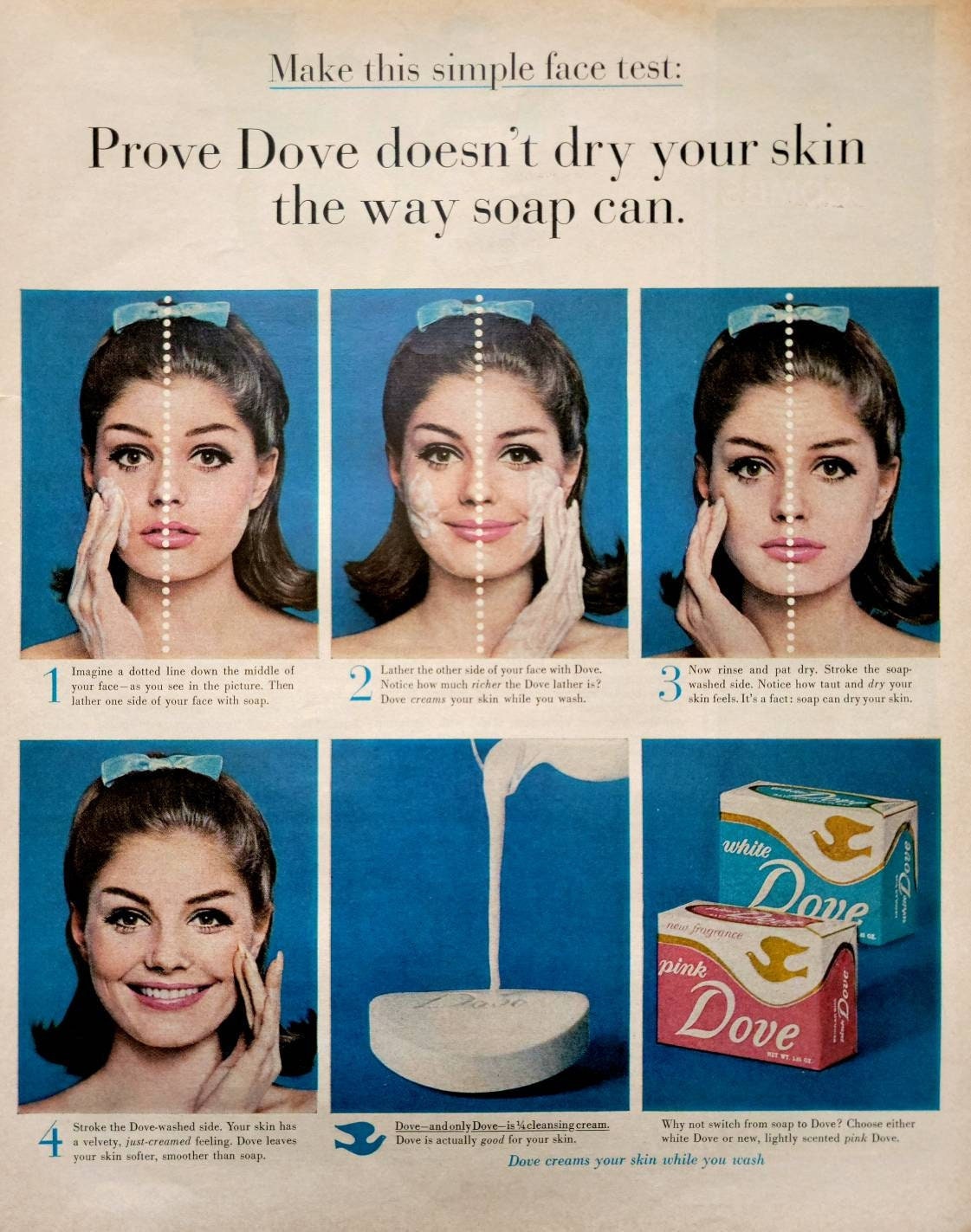This vintage advertisement poster has a charming sepia tone, emphasizing its nostalgic allure. The background of the page is light pink, and at the top, in bold black letters, it instructs readers to "make this simple face test." Underneath this, a teal-colored horizontal line separates the introduction from the main content, reiterating in black text, "prove Dove doesn't dry your skin the way soap can."

The ad is divided into six sections, each with accompanying text in black, though some parts are difficult to decipher. Below the headings, six images are arranged horizontally. The first four images sequentially depict a young woman with short, shoulder-length black hair adorned with a blue hair ribbon. Her face is split down the middle by a vertical white dotted line. In these images, she demonstrates a skincare test by applying soap on one half of her face and Dove on the other. The sequence demonstrates the differences these products have on her skin:

1. **Image 1:** Accompanied by the text, "Imagine a dotted line down the middle of your face. Then lather one side of the face with soap."
2. **Image 2:** Reads, "Lather the other side of the face with Dove. Notice how much richer the Dove lather is. Dove cleans your skin while you wash."
3. **Image 3:** Says, "Now rinse and pat dry. Stroke the soap-washed side. Notice how taut and dry your skin feels. It's a fact. Soap can dry your skin."
4. **Image 4:** Conveys, "Stroke the Dove-washed side. The skin has a velvety, just-cream feeling. Dove leaves your skin softer, smoother than soap."

In the fifth image, the transformation shifts from testimonials to branding, showing milk being poured over a bar of Dove soap accompanied by a logo of a dove in blue. The caption states, "Dove and only Dove is 1/4 cleansing cream. Dove is actually good for your skin."

The final, sixth image, showcases two packages of Dove soap. The top package labeled "White Dove" features a predominantly white design with teal at the bottom, while the bottom package labeled "Pink Dove" combines white at the top with pink at the bottom. The text encourages readers to "switch from soap to Dove" and choose between the scents, concluding with, "Dove creams your skin while you wash."

Overall, this meticulously detailed ad underlines Dove's ability to keep skin softer and smoother compared to ordinary soap, thanks to its unique formulation.